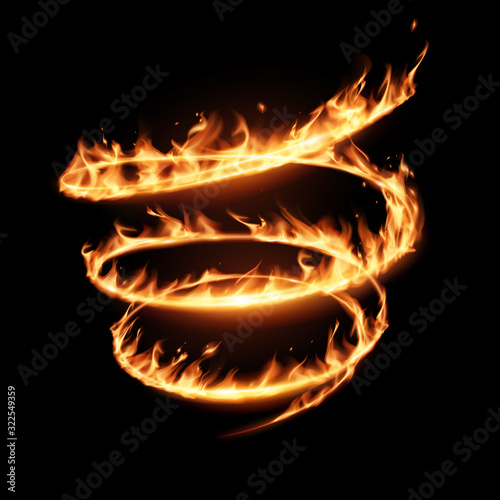The image features a dramatic black background overlaid with faint, diagonal gray text repeatedly stating "Adobe Stock" to indicate copyright. The central focal point is a mesmerizing spiral of fire, vividly depicted in orange and yellow hues, starting from the upper right corner and swirling towards the left, looping around four times before ending towards the bottom center. This thin, interconnected spiral of fire, about a half-inch thick, features short, bright flames shooting upward from each loop. The background remains predominantly black, enhancing the vibrancy of the fiery swirl. In the lower left-hand corner, vertically written text reads "Adobe Stock," followed by a vertical line and the number "3-2-2-5-4-9-3-5-9."